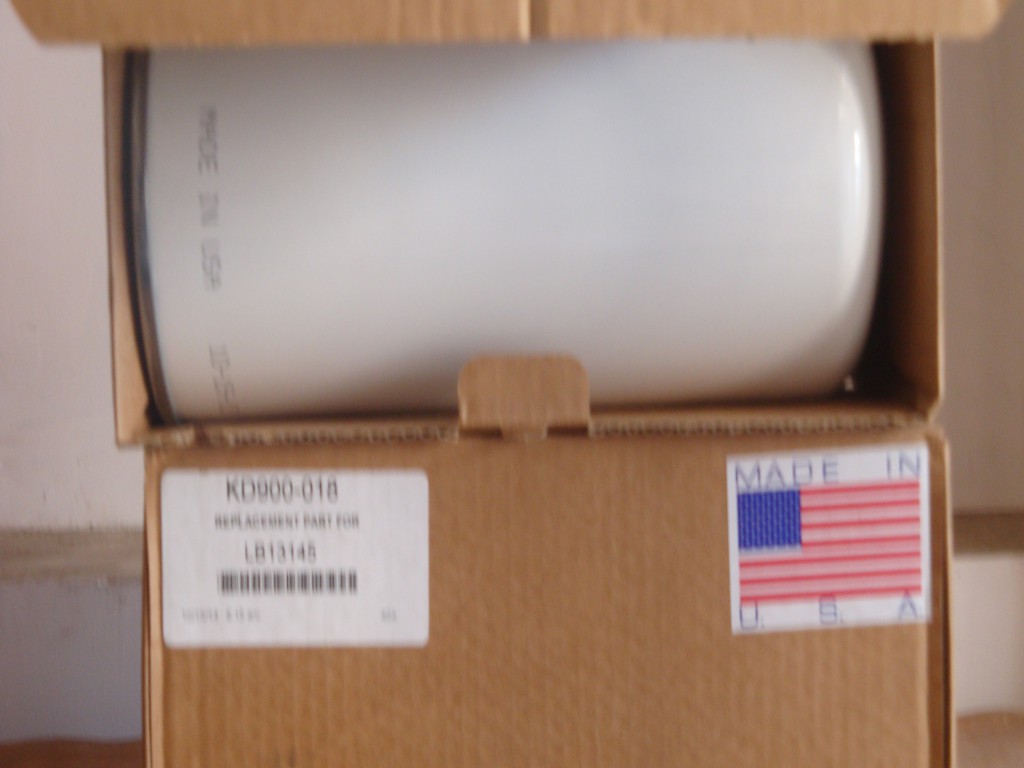A rectangular, light brown cardboard box sits open on a light cream-colored table. The box features two side panels for easy opening. On the upper right corner of the lid, a white sticker with blue text reads "Made in USA," accompanied by a vibrant red, white, and blue American flag. The left side of the box displays a sticker that reads "KD900-018 Replacement Part for LB314S," along with a somewhat blurry barcode. Inside the box, there is an off-white cylindrical metal object, likely an oil filter for a car, adorned with numbers across its bottom.